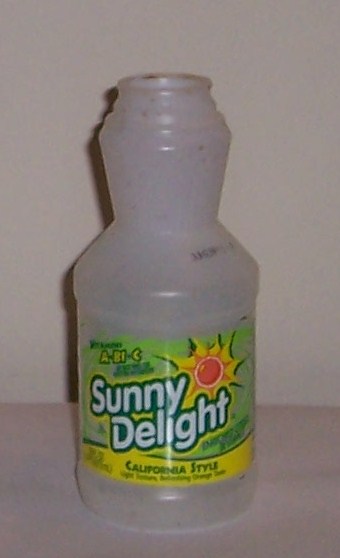The image features an empty Sunny Delight plastic bottle set against a gray background. The bottle itself is white with a prominent green label. The front of the label displays the brand name "Sunny Delight" in large white letters, outlined in green. There's a bold red sunburst graphic with yellow rays radiating from the center. At the bottom of the label, a yellow strip contains the text "California Style" in green letters. The label also highlights the vitamins A, B, 1, and C, indicated in green and yellow letters. Additionally, a small black date stamp is visible on the side of the bottle.